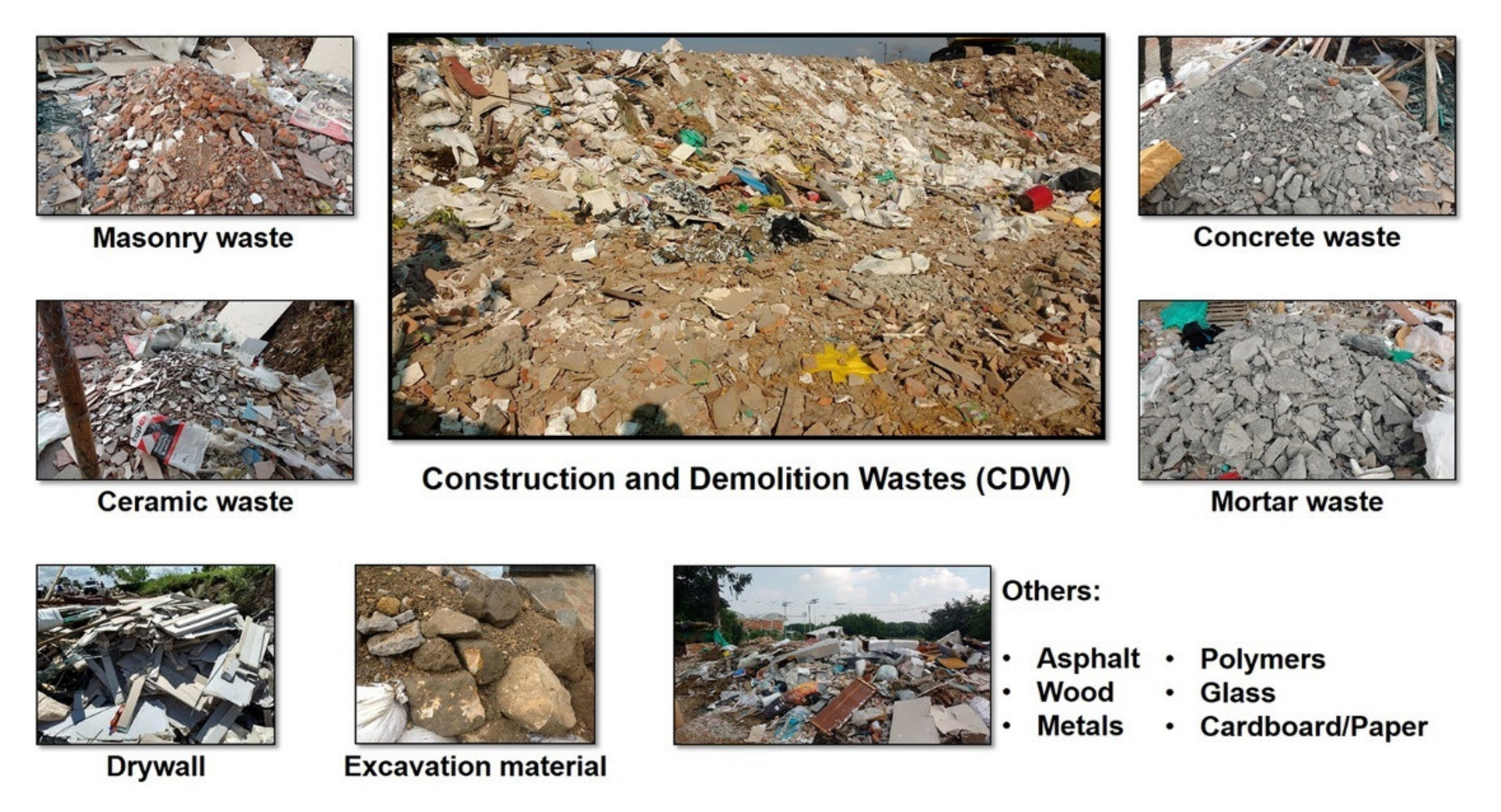This digital art image serves as a detailed diagram of various types of construction and demolition wastes, collectively abbreviated as CDW. The composition is set against a white background and features a centrally positioned larger photograph captioned "Construction and Demolition Wastes (CDW)." Surrounding this central image are eight smaller rectangular photographs, each accompanied by descriptive text.

Starting from the top left, we see:
1. **Masonry Waste** - Characterized by brownish-red debris.
2. **Ceramic Waste** - Identified by its predominantly white fragments.
3. **Drywall Waste** - Comprising slats of wood stacked in piles.

On the bottom row, spanning horizontally across the image:
4. **Excavation Material** - Large, variably shaded brown stones.

To the right, we find:
5. **Concrete Waste** - Smaller gray slabs.
6. **Mortar Waste** - Similar to concrete waste but slightly larger in size.
7. **Other Wastes** - A mixed collection visually represented, with bullet points listing asphalt, wood, metals, polymers, glass, cardboard, and paper.

This thorough depiction provides an educational look at the variety of waste materials produced during construction and demolition processes.